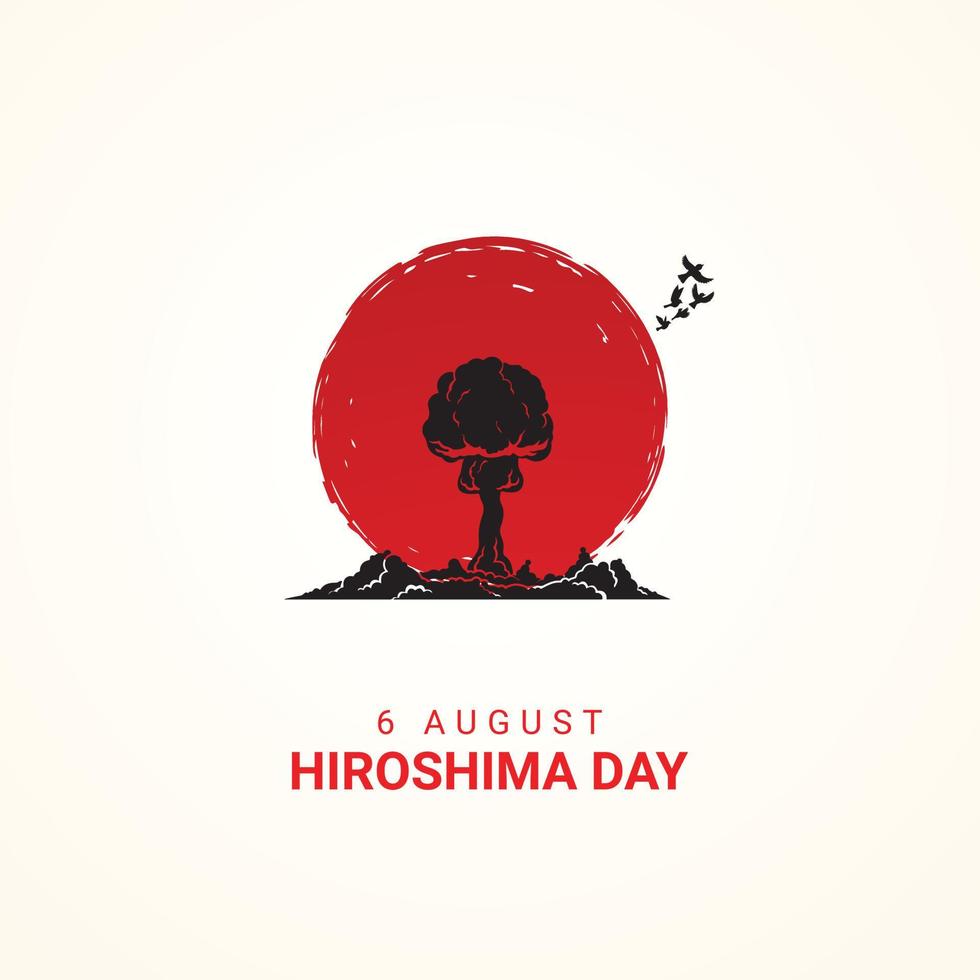The image depicts a poignant, stylized tribute to Hiroshima Day, captured in a monochromatic palette with a bold red accent. Set against a stark black-and-white background, a large red circle dominates the composition, reminiscent of the Japanese flag but with added symbolic elements. Inside the red circle, a detailed black illustration of a mushroom cloud represents the devastating atomic bomb explosion. Above the cloud, small black birds are depicted flying away, enhancing the sense of aftermath and loss. The red circle itself is not solid; it appears textured, almost as if sketched with a pencil, and contains a few subtle white lines. Beneath this powerful imagery, the text "6 August Hiroshima Day" is prominently displayed in red, with the date "6 August" rendered in a slightly smaller, thinner font than the rest. The image is minimalistic yet striking, designed to evoke reflection and remembrance of the tragic event.